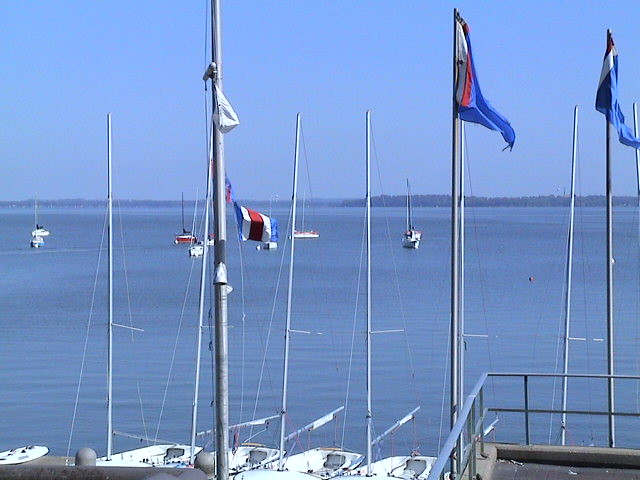The photograph depicts a serene marina scene. In the foreground, a concrete sidewalk with a metal railing provides vantage for the photographer, overlooking a collection of docked sailboats. These sailboats, predominantly white with long tall masts some adorned with blue, white, and red flags, stand prominently. Notably, there's a blue and white flag on the right side of the scene, while centrally, a smaller red, white, and blue flag is visible. Some masts carry triangular wire frames, typical of sailboats, though most lack raised sails. 

At a lower level beyond the railing, a few sailboats rest calmly in the tranquil, bluish-gray water, with only slight ripples disturbing the surface. Further out, five small boats mirror those docked nearby, with one notable red boat adding a splash of color. Background elements reveal hazy blue mountains to the right and a distant shoreline straight ahead, which appears faint but lined with small structures or possible trees. The sky, entirely cloudless, completes the picture with its consistent, slightly overcast blue hue, while a potential lighthouse punctuates the horizon, blending into the overall blue theme of the image.